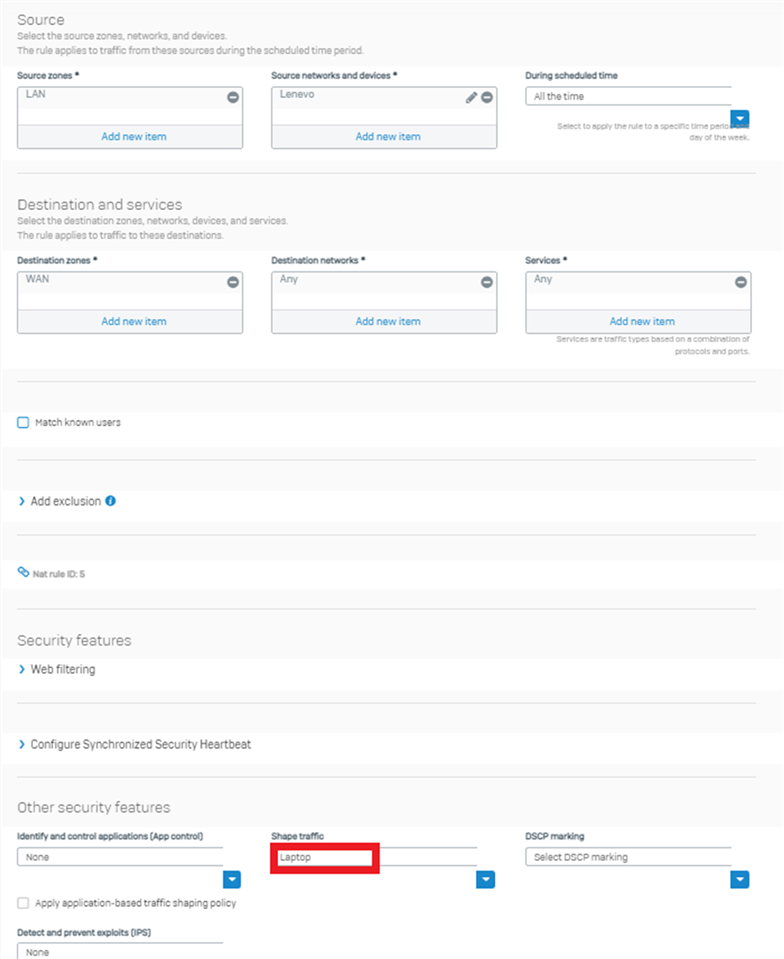This image features a detailed interface primarily set against a white background. At the very top, there is a gray bar titled "Source," accompanied by an instruction to "Select the source zones, networks, and devices. The rule applies to traffic from these sources during the scheduled time period."

Beneath this header is a structured layout with several labeled boxes:
1. On the left, a box titled "Source Zones" contains the designation "LAN."
2. To its immediate right, another box labeled "Source Networks and Devices" is marked "Lenovo."
3. Further to the right, a section specifies the scheduling, labeled "During scheduled time," and reads "All the time."

Directly below this section, a new category titled "Destination Services" instructs users to "Select the destination zones, networks, devices, and services. This rule applies to traffic to these destinations."
1. On the far left within this category, a box labeled "Destination Zones" shows "WAN."
2. To its right, a box titled "Destination Networks" reads "Any."
3. Next to this, the final box in the row, labeled "Services," also reads "Any."

Following these boxes, there are textual lines that include:
- "Match known users"
- "Add exclusion"
- "Rule ID 5"

The next section, labeled "Security Features," lists several specific functionalities:
- "Web filtering"
- "Configure synchronized security heartbeat"
- "Identifying and controlling applications"
- "Shape traffic"
- "DSCP marking"
- "Apply application-based traffic shaping policy"
- "Detect and prevent exploits"

The interface is designed to provide a comprehensive selection of source and destination criteria along with multiple security features for configuring traffic rules.